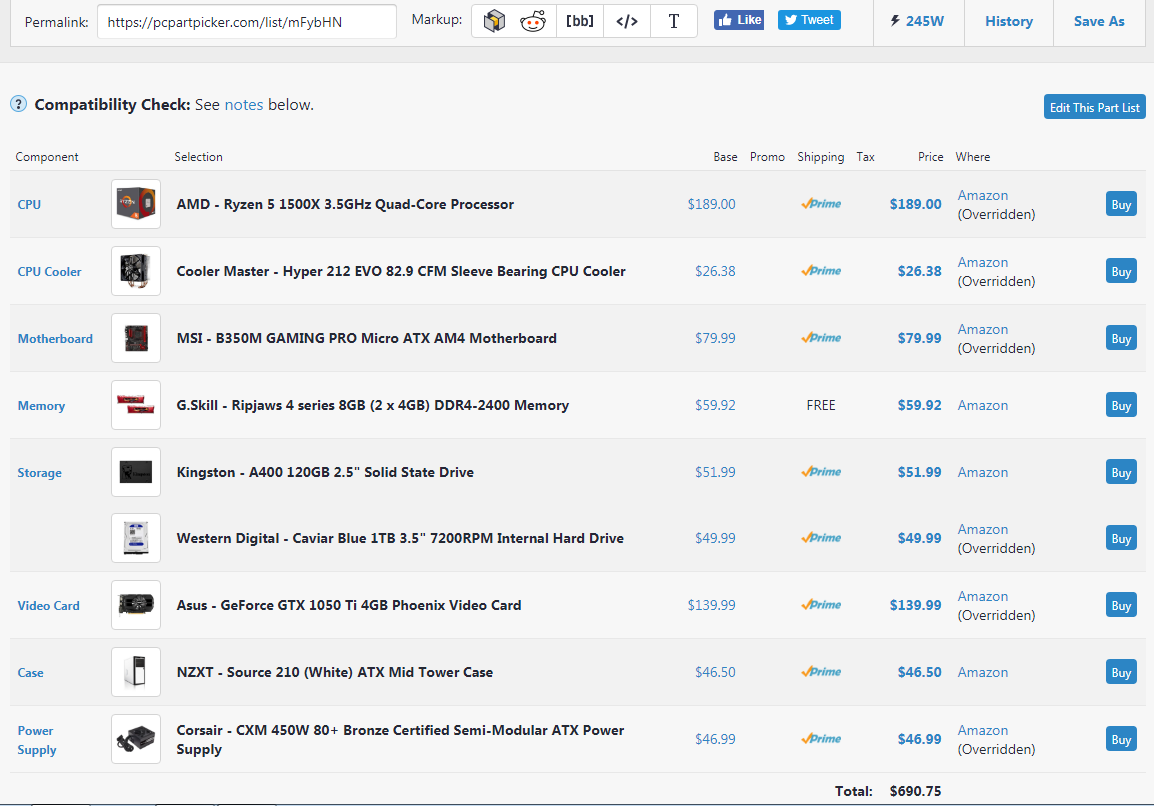Screenshot of the website "PCPartPicker.com":

The webpage features a pristine white background adorned with blue and black text, complemented by a variety of icons representing different components. At the top of the page, there is a clear horizontal navigation layout with categories such as: 

- Compatibility Check ("See notes below")
- Components
- Selection
- Base
- Promo
- Shipping
- Tax
- Price
- Where

Under the "Components" section, the list includes essential parts like:

- CPU
- CPU Cooler
- Motherboard
- Memory
- Storage
- Video Card
- Case
- Power Supply

Each component has a corresponding image displayed to the right. Moving to the "Selection" category, it lists product names like:

- AMD
- Cooler Master
- Kingston
- Western Digital
- Asus

Next, the "Base" category presents prices in blue text, followed by the "Promo" section, which indicates that there are no current promotions. In the "Shipping" category, all items are marked as "Check Prime" except for the memory, which is listed as free shipping. The "Tax" field remains blank. The "Price" category reveals individual prices in bold blue text, and the total cost for all selected items is prominently displayed as $690.75. Finally, the "Where" category specifies the retailer, with "Amazon" appearing in blue text for each item. On the far right, there are blue squares with "Buy" written in white text inside them, indicating purchase options for each product.